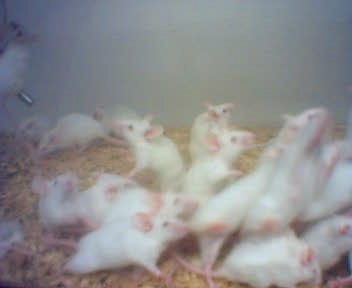The photograph captures a group of white lab mice with red eyes and pink features, including ears, legs, and long tails, situated in a glass tank. The mice are energetically congregating towards the bottom-right corner of the tank, presumably drawn by the presence of food. They are on a bed of beige mulch or wood shavings that lines the bottom of the tank. The background is subtly gray, and the image is slightly out of focus, offering a somewhat blurred perspective. A silver water spout, presumably part of a feeding bottle, is noticeable in the top left corner of the tank. The mice appear to be densely bunched together, with some scattered towards the left and back of the tank, suggesting a lively and curious atmosphere.